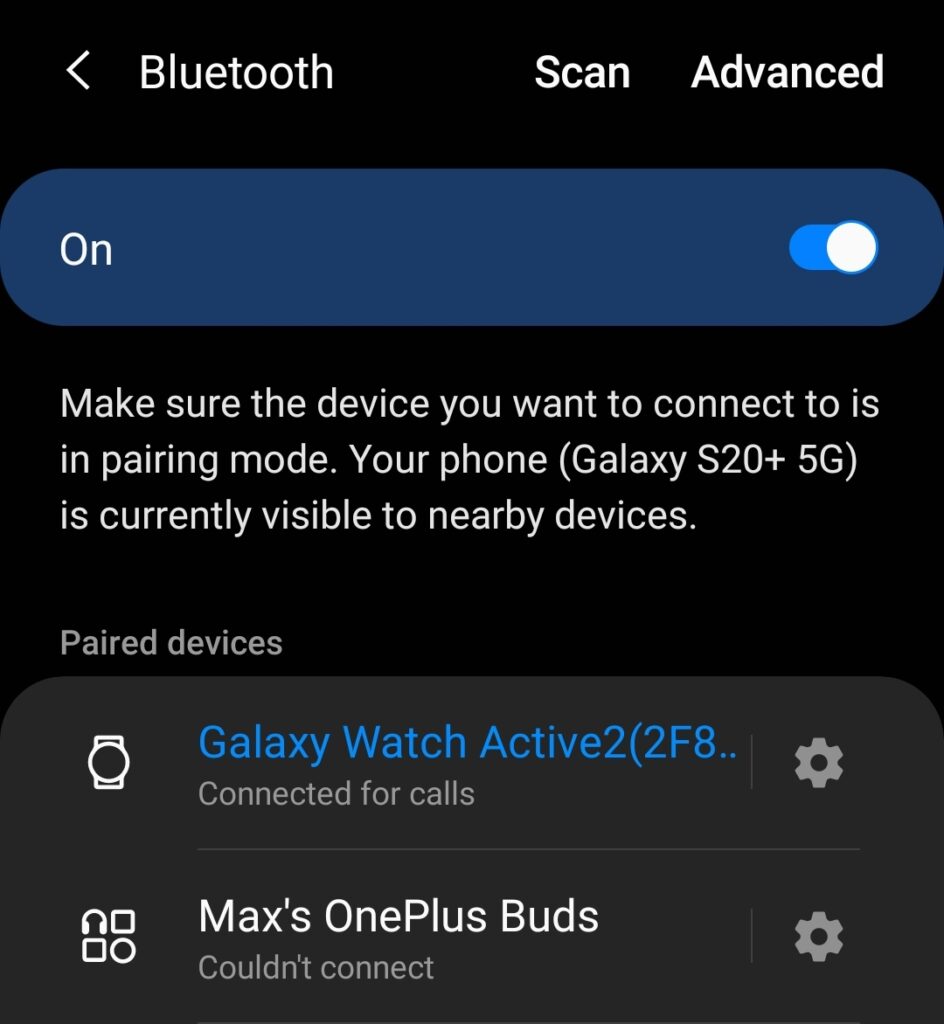Here's a refined and detailed caption for the image described:

---

Screenshot from an Android device in dark mode. The background is black. At the top of the screen, there is a left-pointing arrow next to the word "Bluetooth" in white text. To the right, there are two options: "Scan" and "Advanced," both highlighted slightly brighter than "Bluetooth."

Below this, in a blue elongated elliptical button with white text, it indicates "ON," showing that Bluetooth is activated, with the switch toggled to the right. 

Directly beneath the button, instructions in white text read: "Make sure the device you want to connect to is in pairing mode. Your phone (Galaxy S20 plus 5G) is currently visible to nearby devices."

Following this, a section titled "Paired devices" appears in smaller white letters. The first paired device is indicated by a watch icon and labeled "Galaxy Watch Active 2, S2F8" in blue text, followed by an ellipsis "...". Below this, it states "Connected for calls" with a settings icon located towards the right.

The next device has a headphones icon, labeled "Maxis One Plus Buds" in white text, with a status message "Couldn't connect" and accompanied by a settings icon.

---